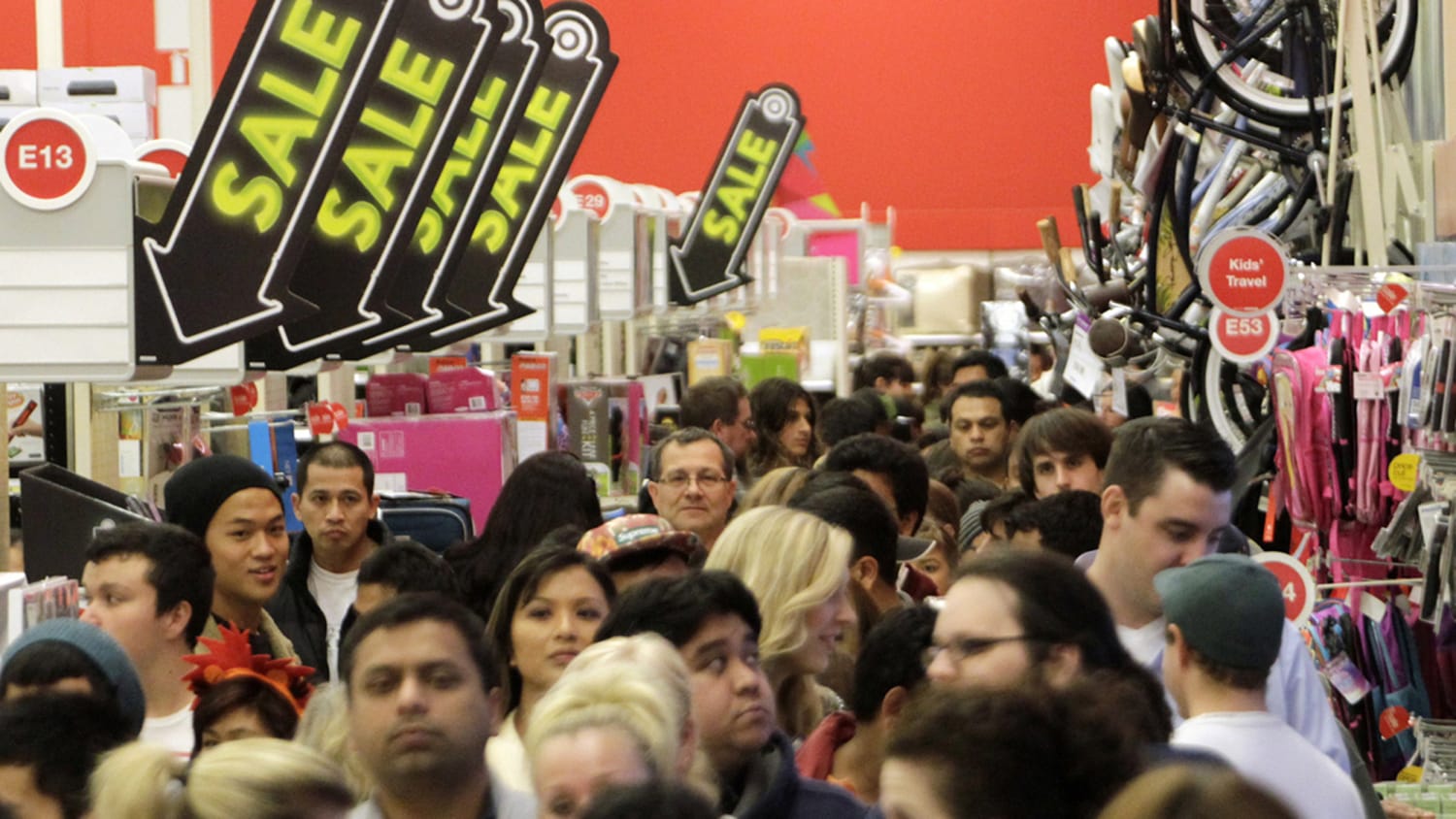This image captures a bustling discount or department store during a sale event. A diverse crowd, comprising men and women of different ages, nationalities, and skin colors, fills a single aisle, moving towards the camera. Among them, various hairstyles such as black and blonde hair, short hair, and individuals wearing caps and beanies are visible. The store's bright red walls dominate the background, giving a vibrant touch to the scene. Suspended vertically on the right side of the aisle are bicycles, with a rack below featuring blue, pink, and red backpacks under a sign that reads "kids travel." On the left, four prominent black signs with white borders and yellow "sale" letters point downwards. Additional markers like "E53" and "E13" help navigate the store, though some numbers are blurred. The crowd, reflecting a mix of styles and appearances, suggests a typical middle-American setting, though the scene's diversity makes it universally relatable.